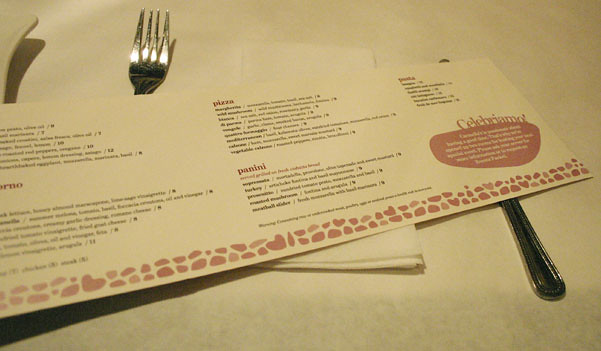A delicate menu rests atop a neatly arranged setup of utensils and a napkin, all placed on a stylish tablecloth. An elegant white image, possibly a decorative light fixture, casts a shadow on the fabric, adding a soft ambiance to the scene. The menu, designed as a slender strip of cardboard, hints at a simple yet authentic Italian dining experience, listing items such as pizza, paninis, and pasta. The name "Celebriano" is prominently featured in the right corner, suggesting it could be the restaurant's name. Most of the menu details remain obscured, adding a hint of mystery. Shadows from the fork and knife play across the tablecloth, with the knife positioned slightly lower than the fork, adding to the overall aesthetic appeal. The partially visible menu and elegant table setting evoke a sense of intimate, casual dining.